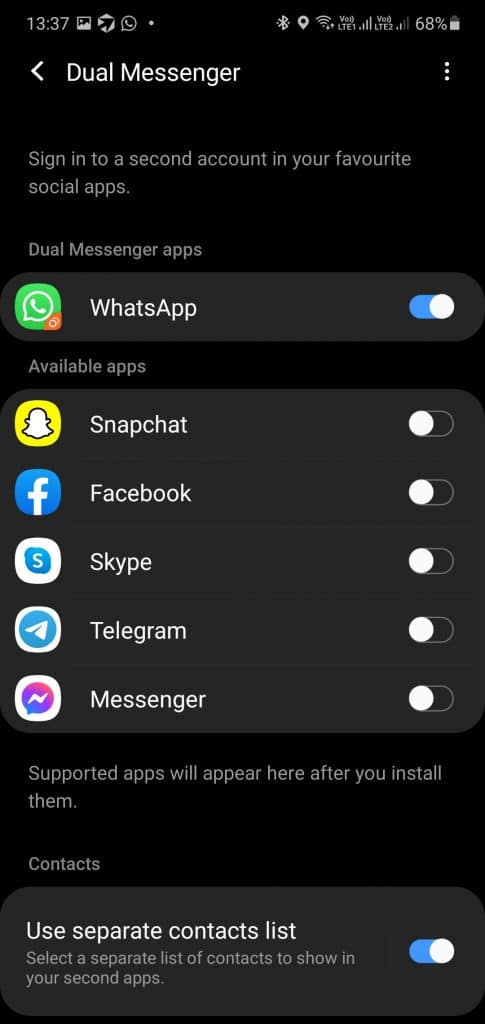This image is a detailed screenshot from a smartphone utilizing dark mode, featuring a black background. At the upper-left corner, the time displays 13:37, indicating the use of a 24-hour clock format. In the upper-right corner, the battery icon shows a 68% charge next to the icons for wireless connection and Wi-Fi.

Beneath this top header, against the black background, white text reads "Dual Messenger," accompanied by a white arrow pointing to the left. Below this, in a light gray font, yet still readable, is a message stating, "Sign in to a secure account in your favorite social apps."

The screen then lists various social media apps, each name written in white text and accompanied by their respective logos on the left. The listed apps and their logos include:
- WhatsApp with its green logo
- Snapchat with its yellow logo
- Facebook represented by a blue circle with a white 'F'
- Skype with the letter 'S' surrounded by a blue circle
- Telegram, featuring a blue logo with a white arrow-like symbol
- Messenger, marked by a purple logo with a white squiggle.

At the very bottom, in white text, it states, "Use separate contact lists," followed by an option to "Select a separate list of contacts to show up in your second apps."